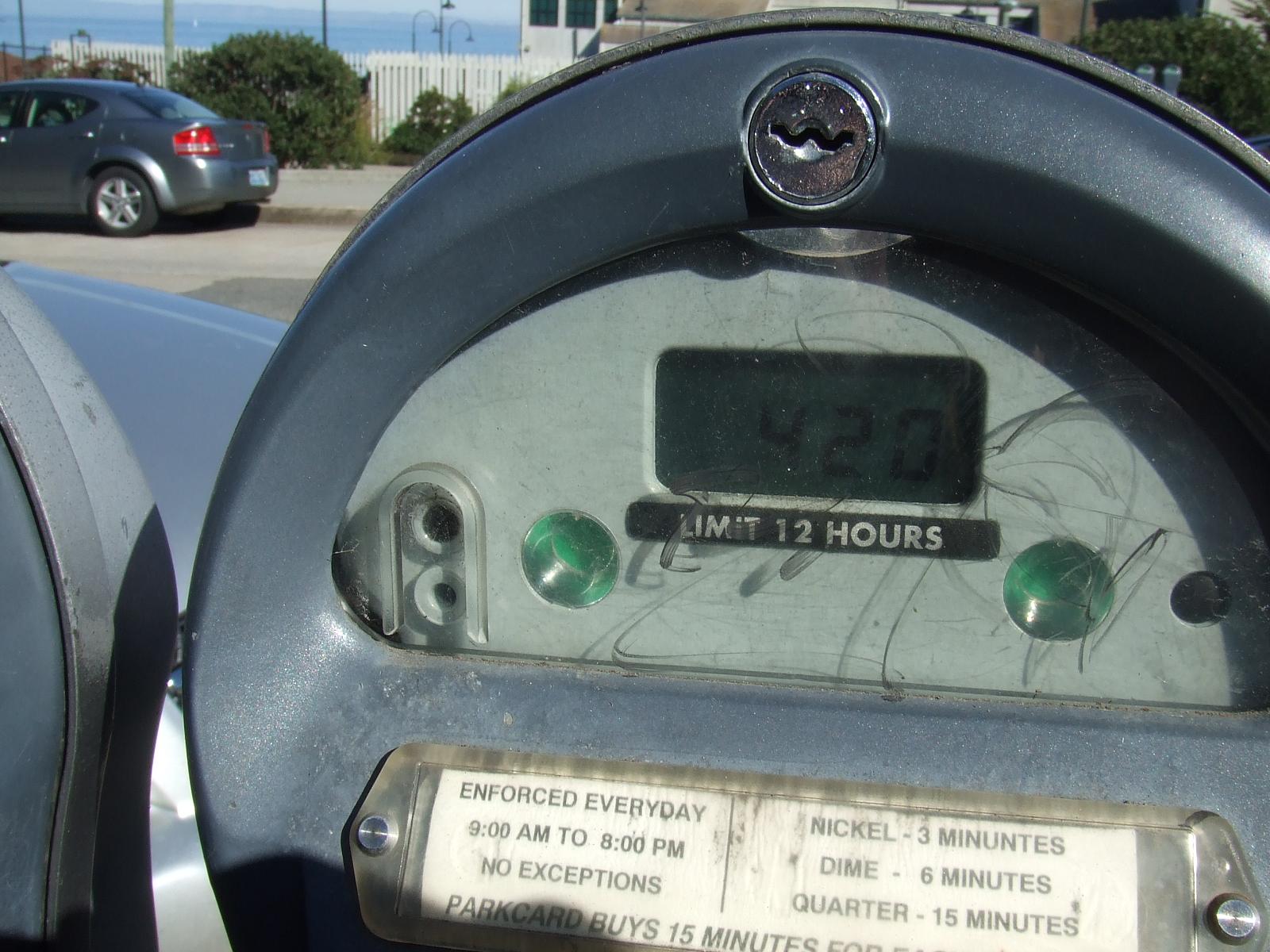This image is set outdoors and features a detailed close-up of a parking meter. The parking meter displays "4-2-0" and states a limit of 12 hours. Beneath these numbers, a small white sign outlines the rules: enforced every day from 9 a.m. to 8 p.m. with no exceptions. The rate is specified as three minutes per nickel, six minutes per dime, and fifteen minutes per quarter. In the background on the upper left, a silver-gray car is parked next to a sidewalk curb. The backdrop includes a mountain range in darker blue, under a light blue sky. Nearby, large bushes with bright to dark green leaves rest against a white picket fence. Behind the fence is a tan-colored house. The image captures both the distinct details of the parking meter and the serene outdoor setting.